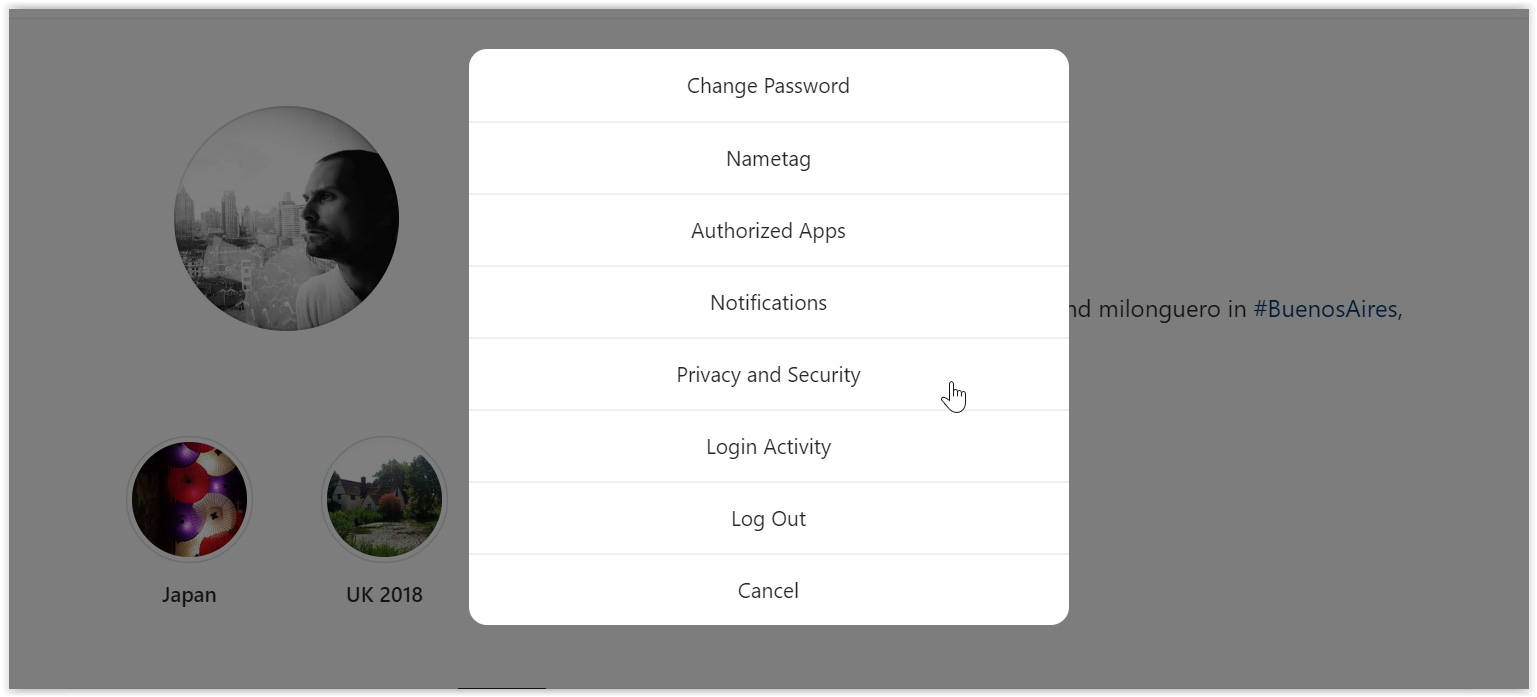The website features a simplistic, minimalist design, devoid of a title or heading, dominated by a medium gray background. Centered on the page is a black-and-white profile picture of a man gazing to his left, set against a cityscape. Below this main image, there is another profile picture, this one related to Japan, featuring purple, white, and red spheres.

Adjacent to the Japan-themed image is another picture labeled "UK 2018," depicting a quintessential British house surrounded by trees. A pop-up window, appearing in the middle of the screen, obstructs part of the background content and is filled with instructions and settings in a gray handwriting-like font. The sections within the pop-up include: Change Password, Name Tag, Authorize Apps, Notifications, Privacy and Security, Login Activity, Log Out, and Cancel.

Partially obscured by the pop-up window, there is additional text that alludes to content behind it, reading "and Milan Guerrero in #BuenosAires," hinting at hidden context and possibly more images or information related to Milan Guerrero. Although the obstructed background elements are not fully visible, their presence suggests further details waiting to be uncovered.